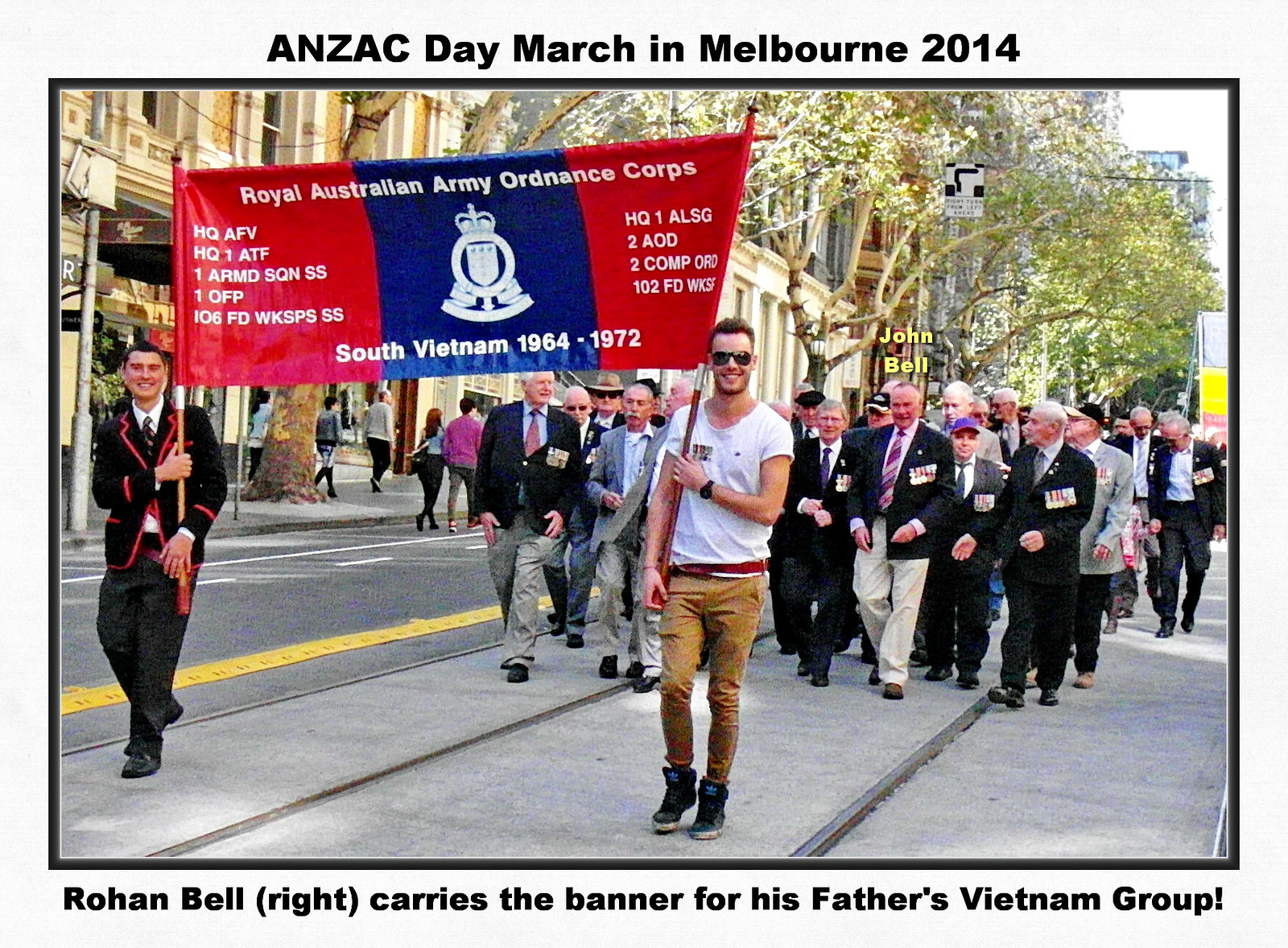This photograph, framed with a light gray border, captures a moment from the ANZAC Day March in Melbourne, 2014. At the forefront, two men—one in a black uniform and the other in a casual shirt with brown pants—proudly hold a vertical red and blue banner of the Royal Australian Army Ordnance Corps. The banner, which features their insignia in the center, reads "Royal Australian Army Ordnance Corps, South Vietnam, 1964-1972." Behind them, a procession of elderly men, adorned in suits and wearing their military ranks and medals, march solemnly. Highlighted amongst them, with his name displayed in yellow text and shadow above his head, is John Bell. The bottom text of the image reads "Rohan Bell, right, carries the banner for his father's Vietnam group." The scene is set against the backdrop of city buildings and trees, capturing the essence of a commemorative parade honoring Vietnam veterans.